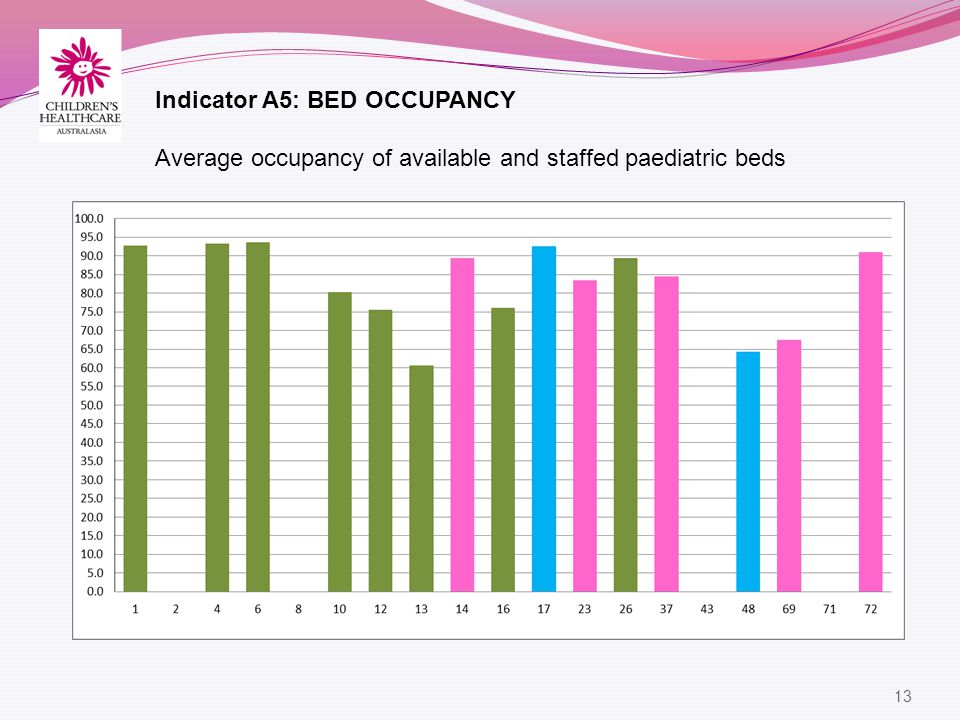The image is a computerized bar graph presented on a landscape slide with a white background and some pink elements at the top. In the top-left corner, there is a logo for "Children's Health Care Australia." Below the logo, the title reads "Indicator A5: Bed Occupancy," with a subtitle that states "Average Occupancy of Available and Staffed Pediatric Beds."

The vertical axis (Y-axis) on the left side of the graph ranges from 0 to 100, with increments of 5. The horizontal axis (X-axis) at the bottom displays numeric labels, but the numbers jump around and are not sequential, listing values such as 1, 2, 4, 6, and 8, continuing up to 72.

The bar graph features bars in different colors (green, magenta, and blue), although there is no legend explaining what these colors represent. For example, the first bar (under the number 1) is green and extends up to approximately 92 or 93. Other key bars are noted as follows:

- Bar 4: Green, approximately 94
- Bar 10: Green, approximately 80
- Bar 12: Green, approximately 76
- Bar 13: Green, approximately 61
- Bar 14: Magenta, approximately 90
- Bar 16: Green, approximately 76
- Bar 17: Green, approximately 93

Additionally, the numbers continue in this non-linear pattern, marking instances such as the 23rd bar being at 85, the 26th at 90, and so forth up to the 72nd bar. The bottom right corner of the slide is marked with the number "13," possibly indicating the slide number.

Overall, this bar graph is used to illustrate the bed occupancy rates across various labels, presumed to be hospital beds, with data points that are differentiated by color but lacking explicit color coding information.